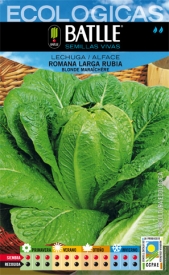The image depicts a seed packet for romaine lettuce, featuring a detailed close-up of a cabbage head with its textured leaves fanning out around the edges. At the top of the cover, "Ecologicas" is written in semi-transparent, low-opacity white type. Directly below this is a black strip with "BATTLE" in bold white letters at its center. Underneath the black strip are three lines of small black text that appear to be names, though they are illegible due to the image size. The bottom section of the cover contains a table divided into four different colored squares, each featuring two rows of dots—three red dots on the top row and three black dots on the bottom row. The background includes a brown wicker basket holding the cabbage and some blue sky with white clouds, adding a natural aesthetic. Additional labels and markings throughout the cover provide further details, but they are too small to decipher clearly.